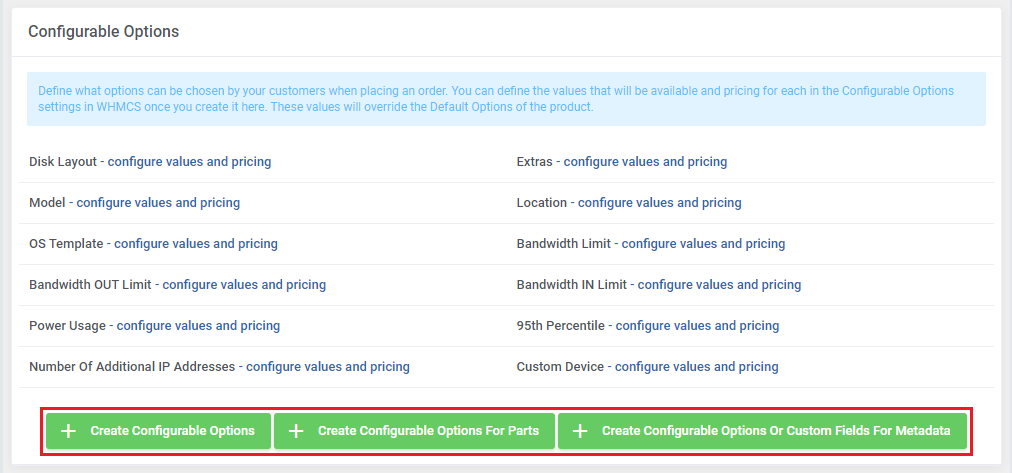The image showcases a website interface related to configuring options for a service. In the upper left corner, "Configurable Options" is prominently displayed in black text. Beneath this header, a blue box with blue text provides instructions: "Define what options can be chosen by your customers when placing an order. You can define the values that will be available and pricing for each in the Configurable Options settings in WHMCS once you create it here. These values will override the default options of the product."

Below the blue box, a list of configurable options is presented in black text. These options include:

- Disk Layout: Configure values and pricing
- Model: Configure values and pricing
- OS Template: Configure values and pricing
- Custom Design: Configure values and pricing
- Domain: Configure values
- Extras: Configure values and pricing
- Location: Configure values and pricing
- Number of Additional IP Addresses: Configure values and pricing
- SSH Public Key: Configure values

On the right side of the interface, the same options are reiterated with prompts to configure values and pricing.

At the bottom of the image, there are three green boxes, each outlined in red, indicating actionable buttons. The first box on the left has a plus sign and reads "Create Configurable Options." The middle box also has a plus sign and reads "Create Configurable Options for Parts." The final box on the right features a plus sign and reads "Create Configurable Options or Custom Fields for Metadata."